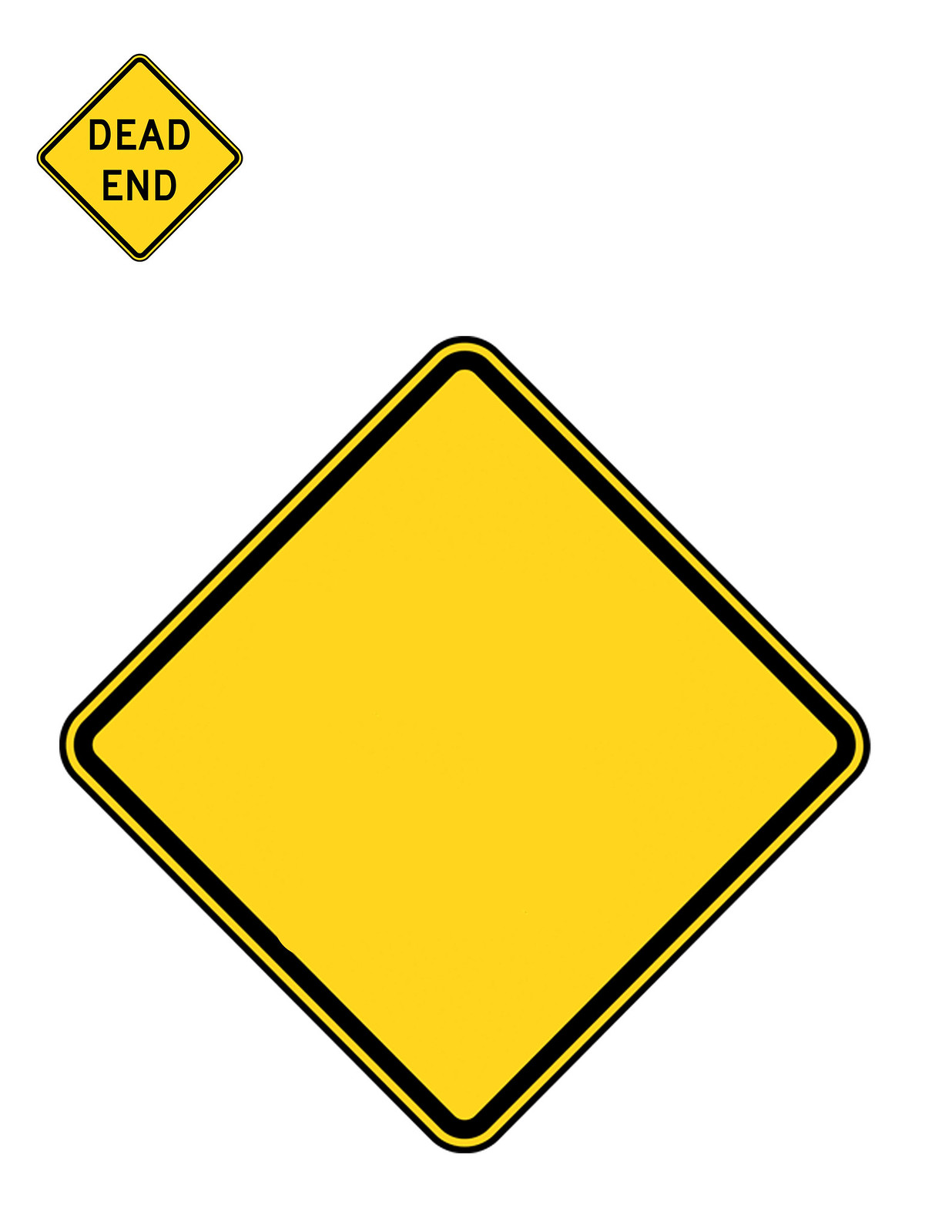Two road signs against a stark white background. The sign in the foreground is a large, gold-yellow diamond with black trim, devoid of any text or symbols. Behind it, a smaller, gold-yellow diamond sign with bold black letters centered in all caps reads "DEAD END." The image quality is exceptionally sharp, with no pixelation, blurring, or color discrepancies. The simplicity and clarity of the composition draw focus exclusively to the two road signs, highlighting their contrasting scales and functions.